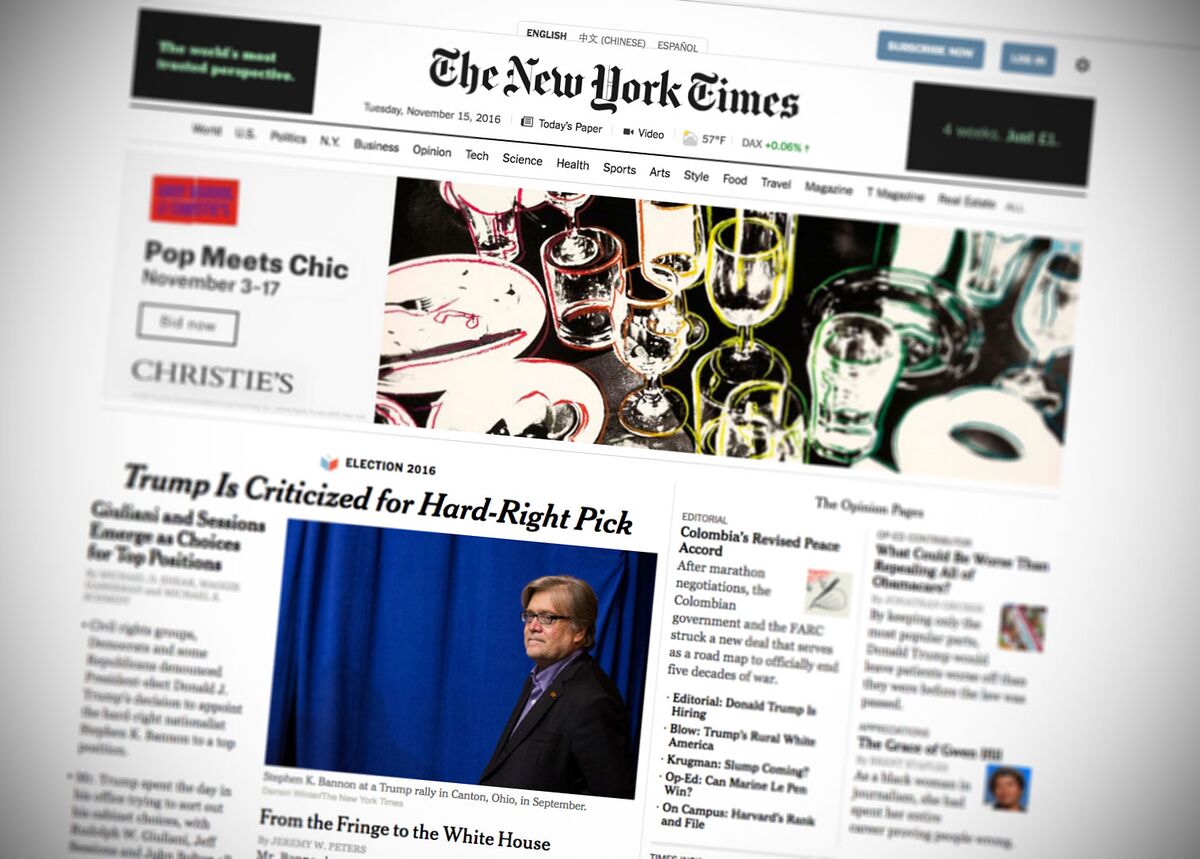Here is a detailed and cleaned-up caption for the described image:

---

A rectangular screenshot captures the front page of The New York Times from Tuesday, November 15, 2016. At the top center, the iconic newspaper's name, "The New York Times," is printed in black italics. Above this title, in small uppercase letters, appear the words "ENGLISH" and "CHINESE," followed by "Espanol" in gray text, indicating the availability of the publication in multiple languages. The date is prominently displayed alongside options for today's paper, video content, and the local temperature.

Beneath a thin black line that spans the width of the page are various categories, laid out from left to right. A noticeable feature is a red rectangular background containing black lettering that reads "POP MEETS CHEEK," abbreviated as PMC. Below this section, there is an announcement for events taking place from November 3rd to 17th.

Further down, a section marked "Christie's" in all caps sits above a large, central photograph that showcases an array of multicolored, clear glasses. Adjacent to this image is a headline concerning the 2016 election: "Trump Is Criticized for Hard-Right Pick," with an accompanying picture of Steve Bannon. Bannon is shown in profile, wearing glasses and a black jacket, against a backdrop of blue curtains.

On the right side of the page, there are several opinion pieces and editorials, including a prominent piece on Colombia's revised peace accord. The article details the Colombian government's new agreement with FARC, as a roadmap to end five decades of conflict. Additional editorial titles appear beneath this article, with various other news stories and images continuing to the right side of the page, some of which are blurred but include visible square-shaped pictures.

---